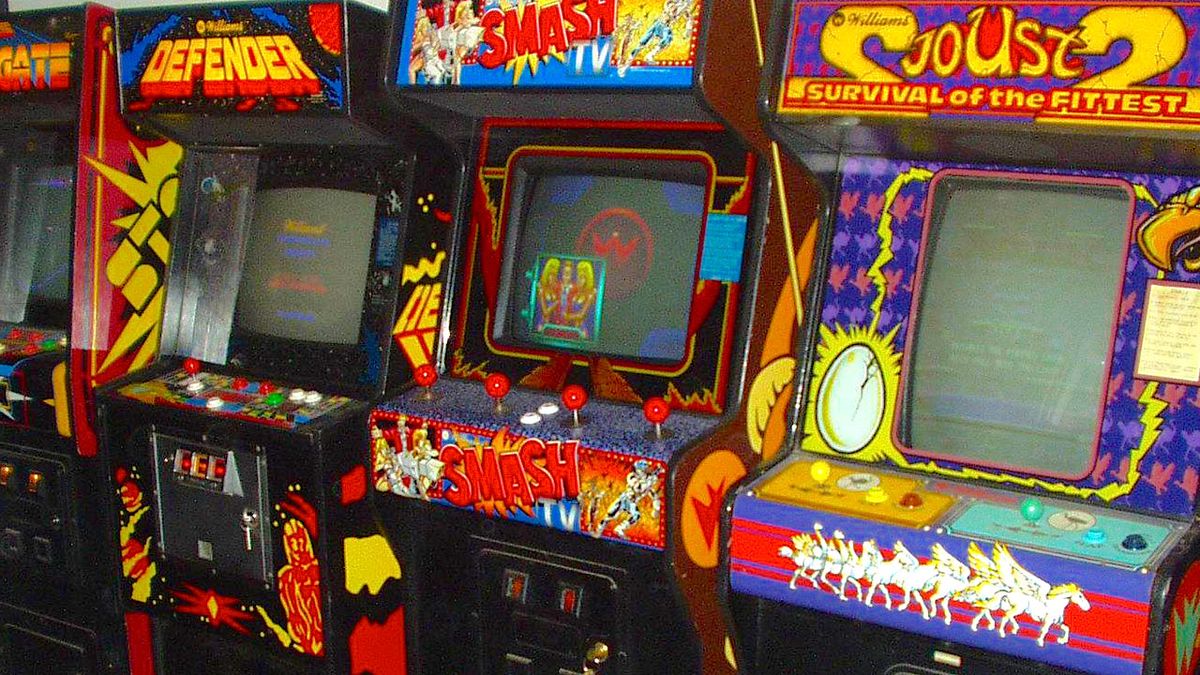This image showcases an arrangement of four classic arcade games from the 70s and 80s, positioned from left to right. From leftmost, only half of the first arcade machine is visible. The second game, "Defender," flaunts a black and blue exterior with red and yellow accents. Its screen is centered, topped with a banner that reads "Defender" in yellow letters, and equipped with red, green, and white buttons, alongside green knobs.

The third arcade machine present is "Smash TV." Its striking design features a screen displaying small images of two blonde women and a man, all encased in a vibrant cabinet adorned with red lettering that says "SMASH TV" at the top, and in white underneath it. This game offers four red joysticks and two white buttons, contributing to its colorful and dynamic look.

Lastly, the rightmost game is identified as "Joust 2: Survival of the Fittest." This machine boasts a fascinating visual with a purple banner, red dots, and prominent yellow lettering. The top features decorative purple and red animals around the central screen. The game includes two uniquely colored joysticks - one yellow and one teal - and accompanying buttons in yellow, teal, dark blue, and red. The front is adorned with purple and red striping, featuring white-winged unicorns.

The games form a slightly angled line from the camera's perspective, with the right side appearing closer than the left. Each arcade machine’s vivid colors of purples, reds, yellows, and blues stand out, capturing the nostalgic essence of vintage arcade gaming.